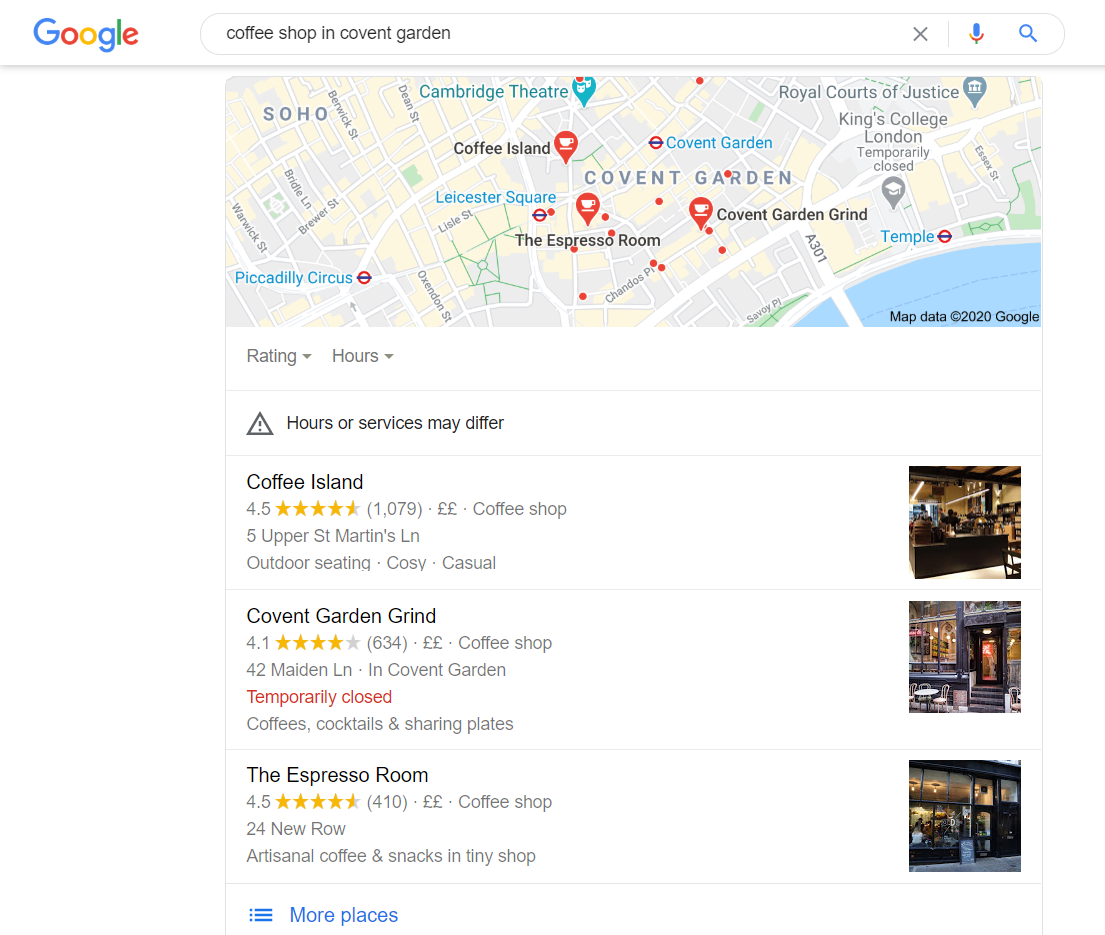A detailed screenshot of a Google search for "coffee shop in Covent Garden" displays various elements. At the top-left, the recognizable Google logo is positioned beside an extended search bar filled with the queried text. To the right of the search bar are an 'X' icon for clearing the search, a blue microphone icon, and a magnifying glass indicating another search bar.

The webpage background is predominantly white, dominated by a large rectangular map at the top of the search results. This map features multiple pin drops marking pertinent locations. Directly below the map, on its left, are two small drop-down menus labeled "Rating" and "Hours". Adjacent to these, a triangle icon precedes a bolded note, "Hours or services may differ".

Beneath the map, the search results appear in a vertical list. Each entry includes the business name, rating, address, and categories on the left, and a square thumbnail image of the business on the right. The first entry is for "Coffee Island", highlighted in bold black font. It has a rating of 4.5 stars out of 1,079 reviews, illustrated by a line of five stars beside the numeric rating and bold text "Coffee Shop". Below the name and rating, the address is displayed, followed by descriptors like "Outdoor Seating" and "Cozy Casual". The remaining results follow an identical format, providing a consistent layout of names, ratings, and thumbnails.